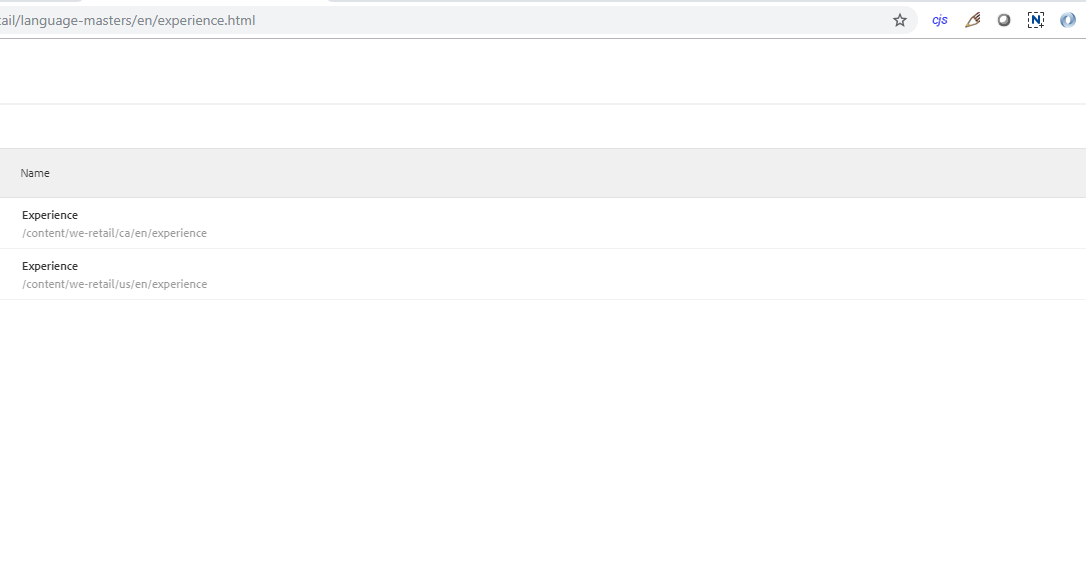The image displays an intricate view of a website's user interface. At the very top, there's a thin horizontal line followed by a gray search bar beneath it. This search bar contains a web address that is partially cut off, showing only a segment of the text. Positioned at the far right end of this search bar is a star icon, indicating an option to bookmark the webpage.

Adjacent to the address bar, there are various icons and text elements including "CJS" and "Blueprint." Additional icons include a pencil, a black circle, a blue 'N' encased in a dotted line and square, and a thicker gray circle, each likely representing different functionalities or navigational aids.

Below this section, the page features a light gray banner with the word "name" aligned to the left in black text. As you move further down, the background turns white, and there’s mention of “experience” in black print, followed by several paths indicating different content locations: 
- "/content/we-retail/CA/EN/experience" 
- "/content/we-retail/US/EN/experience"

These paths are neatly displayed as text lines, one below the other, providing a clear view of site structure and navigation.